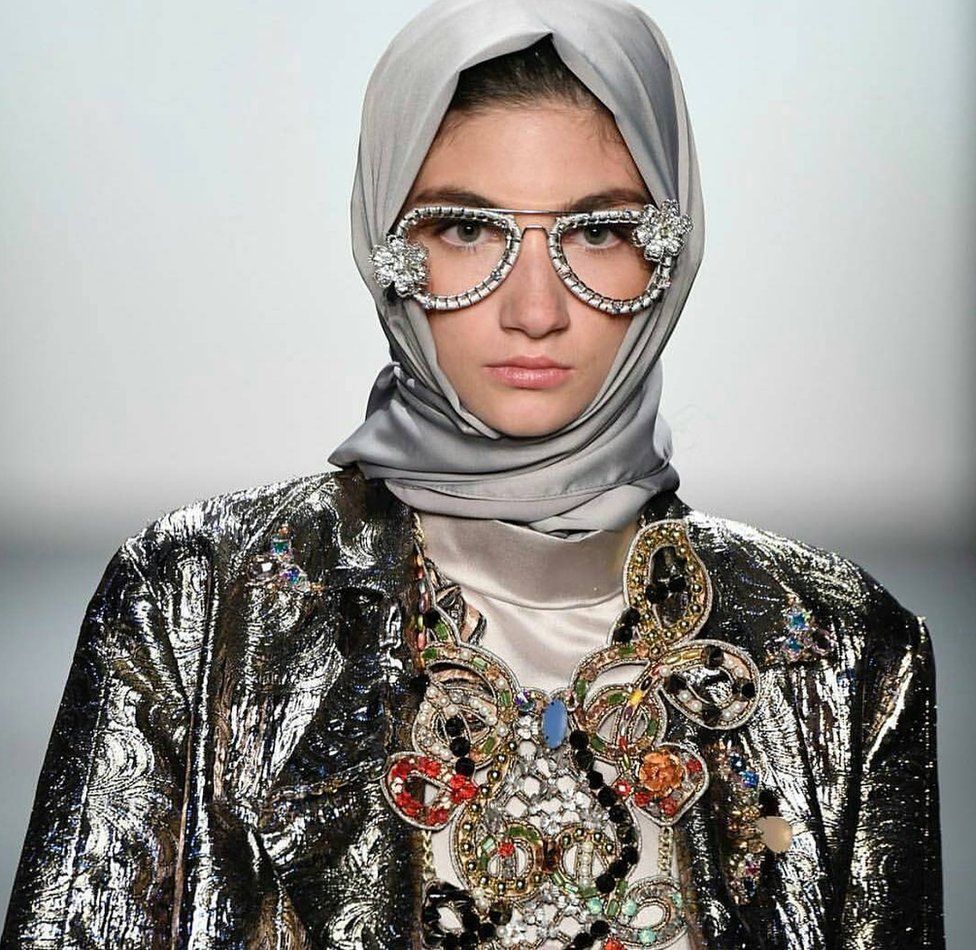In this striking color photograph, a young female model, seemingly on a runway, is showcased in a square format image. She is dressed in a highly avant-garde outfit that captures immediate attention. Her dark hair is pulled back and partially covered by a chic, silver headscarf that wraps under her chin and flows back from her neck. Her neutral expression highlights her dark eyes and well-defined brows, adding to her composed demeanor. 

The model’s glasses are particularly eye-catching, resembling Elton John's classic style but with a contemporary twist: they're crafted from snakeskin and decorated with clusters of diamond-like rhinestones in the shape of flowers at the upper right and lower left corners of the frames.

Her attire includes a luxurious pewter champagne-colored satin turtleneck, topped with a dark metallic, shiny jacket that adds a touch of vintage flair reminiscent of something a grandmother might wear. The most elaborate feature of her ensemble is the massive, intricate necklace she wears. Composed of approximately 20 different pendants, the necklace is a complex weave of black beads and clear stones intertwined with red and gold highlights, creating a visually arresting seal-like piece around her neckline. The overall style of the photo suggests photographic representationalism, merging realism with high fashion photography against a neutral gray background.